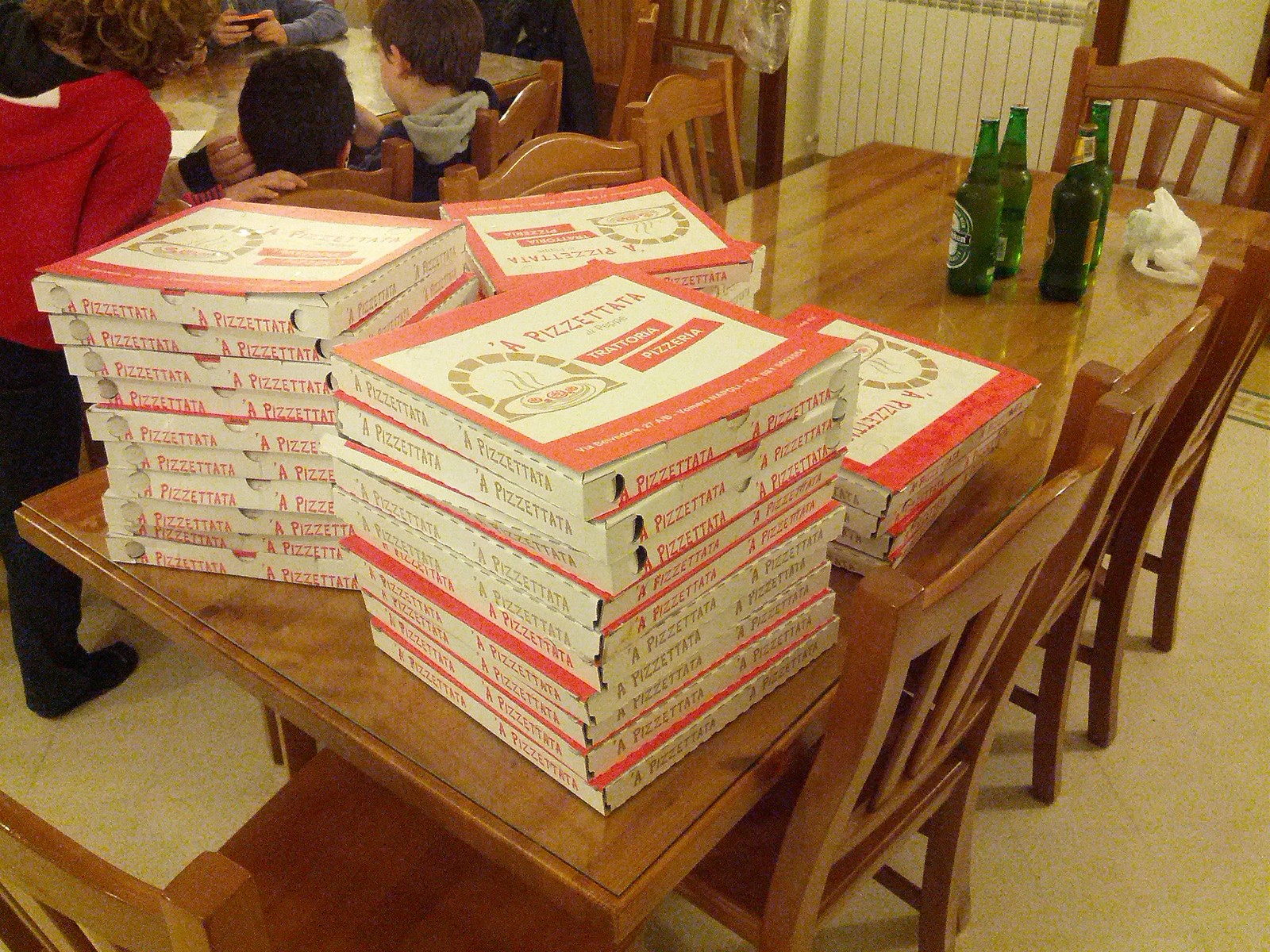The photograph depicts a rectangular wooden dining room table surrounded by eight wooden chairs, arranged with three on each side and one at each end. Dominating the table are four towering stacks of pizza boxes, bringing the total number of boxes to over thirty. The pizza boxes are decorated in red, white, and gold with text reading "a pizza tata," "trattoria," and "pizzeria." The stacks of pizza are positioned toward one end of the table, while at the opposite end, there are four unopened Heineken beers in green glass bottles alongside a crumpled white plastic bag. In the background, partially cropped from the image, are other similar tables with people gathered around them. One person dressed in a red jacket stands nearby, and two children are seated with their backs facing the camera, while another individual’s hands can be seen holding a phone.